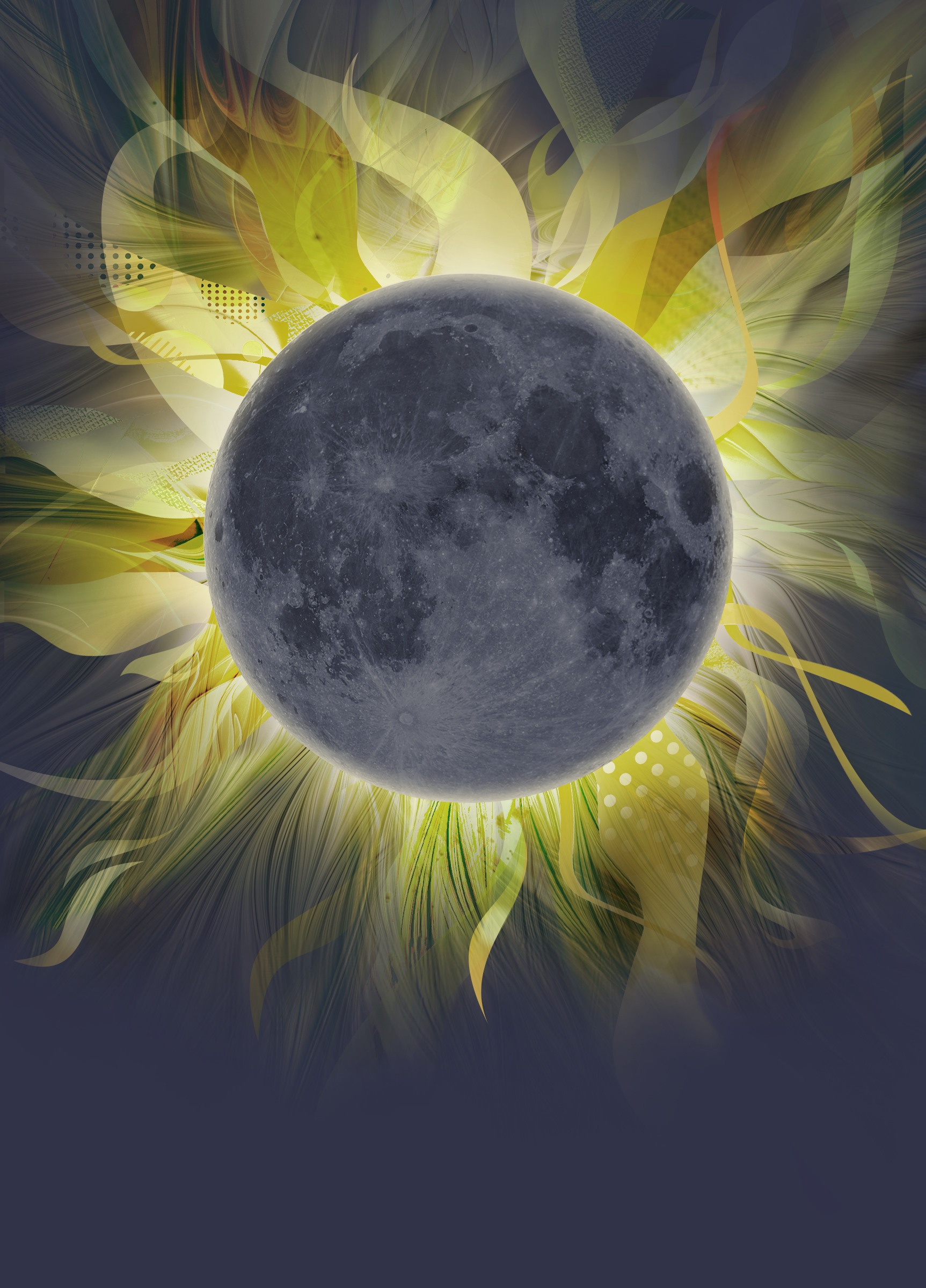In this digitally-constructed image, the central focal point is a large, gray-tinted circle representing the moon, detailed with divots, dark patches, and light marks. Radiating from behind the moon are vibrant, yellow tendril-like projections that encircle it, suggesting the appearance of a glowing halo or a sunflower. These tendrils are adorned with intricate patterns, including dots and varying lines, which add texture and depth to the scene. The backdrop of the image is a dark gray to black, enhancing the luminous effect of the yellow radiance around the moon, giving an impression of the moon glowing against the dark sky. The detailed composition merges elements of nature and abstract art, creating a visually striking and ethereal scene.